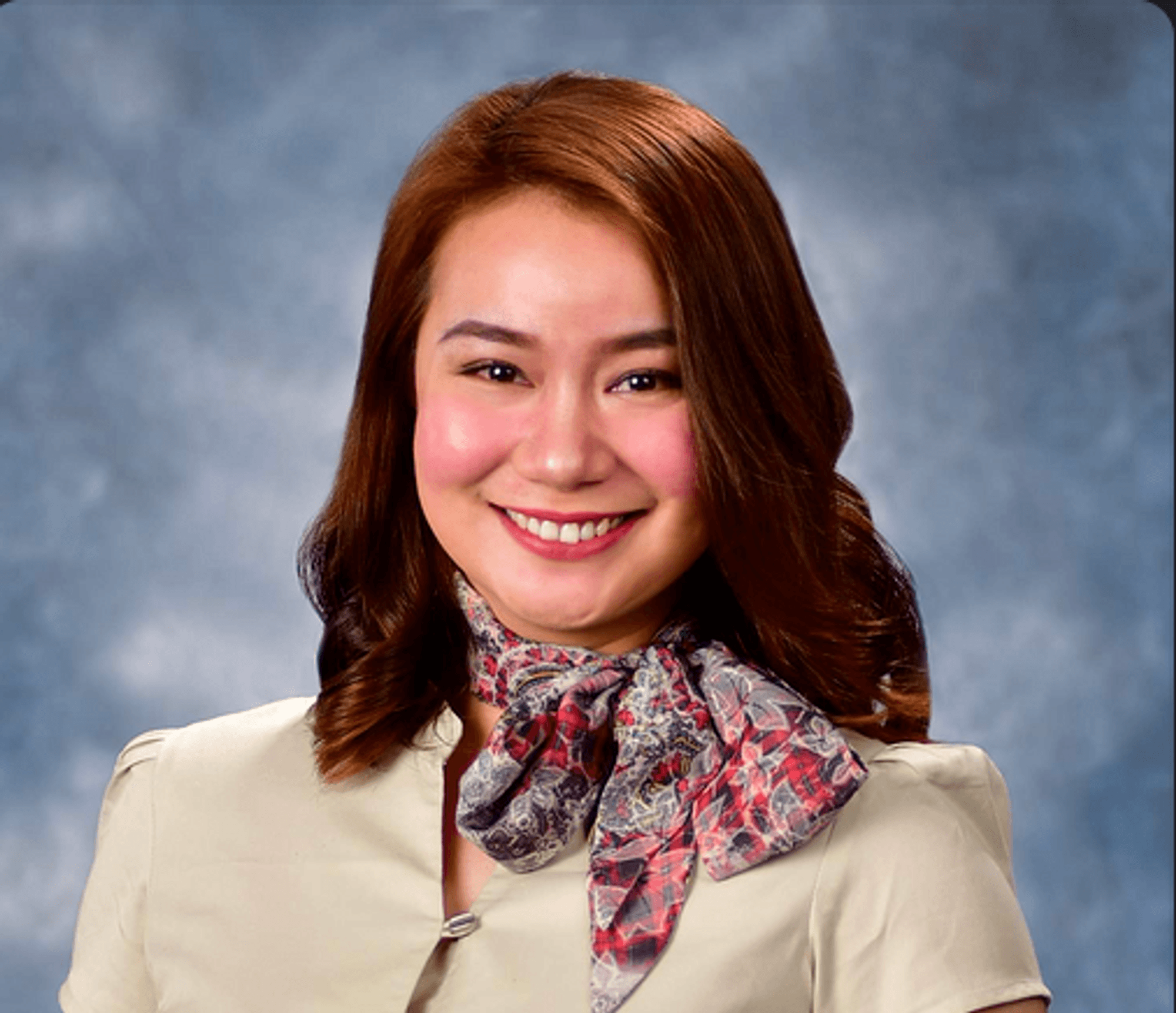In this professional portrait, likely intended for a school or work setting, a smiling young woman with fair skin and a blend of Caucasian and possibly slight Asian features poses against a light blue and white background. Her shoulder-length reddish-brown hair, parted on the right side, is straight at the top and slightly curls at the ends, with some strands resting in front and others in the back. She has rosy cheeks, light red lipstick, and straight, visible top teeth. Her symmetrical facial features include small eyes and a wide base of her nose. She is adorned with a colorful scarf in shades of red, white, and blue, tied in a bow to one side of her neck, and is wearing a tan, short-sleeved blouse or dress that is buttoned up near the top. The portrait crops just above her bosom, emphasizing her cheerful demeanor and professional presentation.